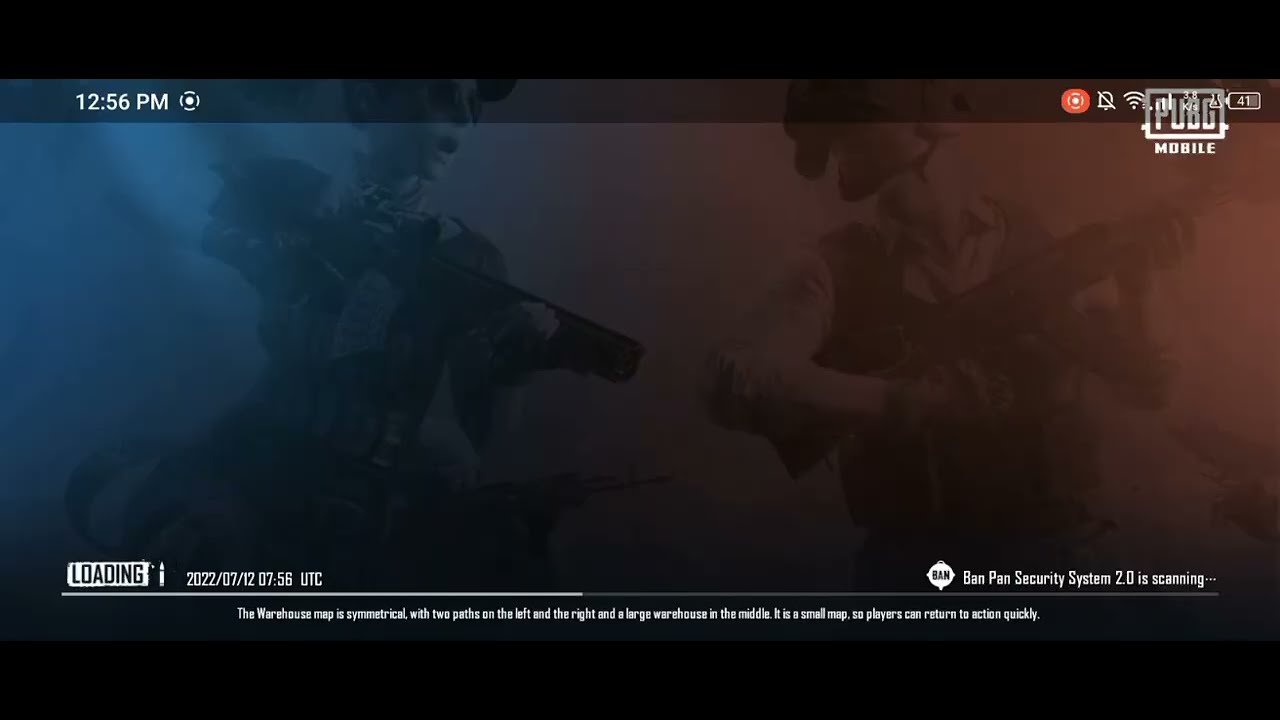This is a detailed screenshot from a mobile game, specifically PUBG Mobile, as indicated in the top right corner. The time in the top left reads 12:56 PM, alongside a red recording dot, and on the top right, the phone's status icons show the battery percentage, a muted notification bell, and a Wi-Fi signal. The bottom of the screen displays "Loading 2022-07-12 07:56 UTC," and a notice about the "BandPan Security System 2.0 is scanning." The middle of the image features a foggy background with two characters: on the left, a punk-styled character holding a sawed-off shotgun with a blue and red design, and on the right, a soldier-like figure holding an automatic weapon. The text overlay describes the warehouse map in the game as symmetrical, with two paths on either side and a large warehouse in the center, emphasizing the map's small size for quick player re-engagement. The colors in the screenshot include black, white, blue, red, orange, and gray, contributing to the overall atmospheric effect of this mobile gaming experience.